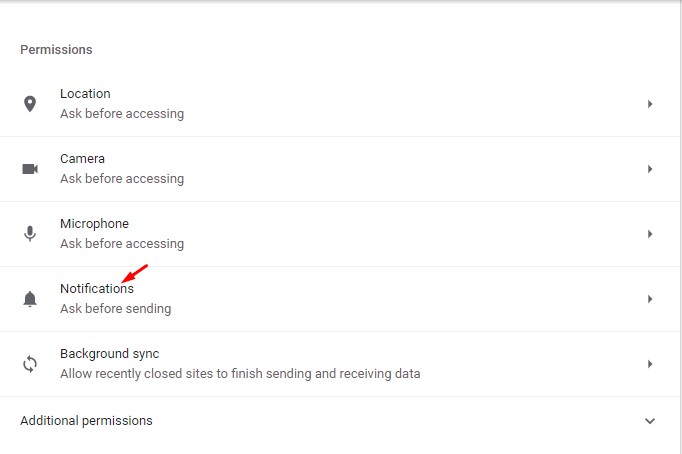This screenshot, likely taken from a smartphone or tablet, captures the permissions page of a settings application. The interface features a simple design with gray text on a white background. The upper left corner succinctly labels this as the "Permissions" page.

The list begins with "Location," identifiable by its pin icon. This entry specifies that the device asks before accessing the location, with an expansion arrow on the right to customize this permission further. Below "Location" is "Camera," accompanied by a camera icon and similar customizable settings for access permissions. The third item is "Microphone," marked with a microphone icon, which also requires asking before access and has an expansion arrow for more options.

The fourth item, "Notifications," is distinguished by an alert bell icon and is highlighted with a prominent red arrow, indicating its significance. This entry handles the permissions for notifications, asking before sending them. 

The final clearly visible item, with a circular icon, is "Background Sync." This option allows recently closed sites to finish sending and receiving data. Like the previous items, it has an expansion arrow for additional settings. Below this section lies an "Additional Permissions" area, which can be expanded to manage further permission settings.